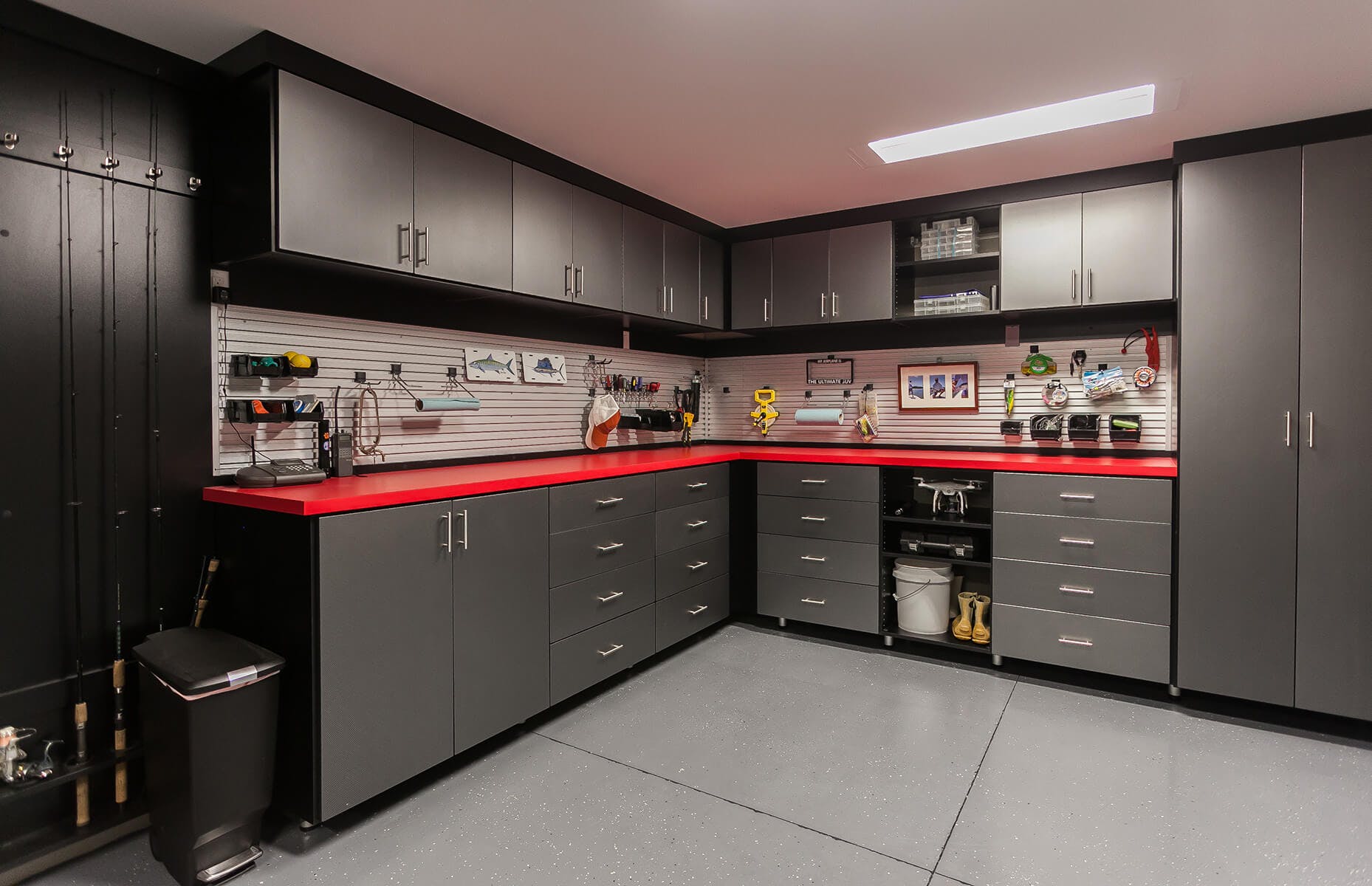The photograph showcases an immaculately organized garage that has been transformed into a functional work area. The garage features a shiny, epoxy-coated tile floor that enhances its clean appearance. The cabinets, all in metallic silver, wrap around one corner of the space, forming an L-shaped configuration. The red countertop on these cabinets is striking and devoid of clutter, emphasizing the high level of organization maintained in this space. Mounted on the wall behind the countertop is a pegboard with a selection of tools and gadgets, neatly arranged but not overly crowded.

Above the pegboard runs an additional row of metallic cabinets, seamlessly matching the lower ones. To the left of the cabinetry, a black trash can is neatly positioned. In an open section at the lower part of the setup, there is a large white bucket and a pair of yellow boots. Additionally, a roll of paper towels is affixed to the wall behind the cabinets for easy access. Various items like fishing lines, garbage cans, signage, and additional buckets contribute to the utility of the space without compromising its tidiness. The entire area appears meticulously swept and free of debris, highlighting its very clean and orderly nature.